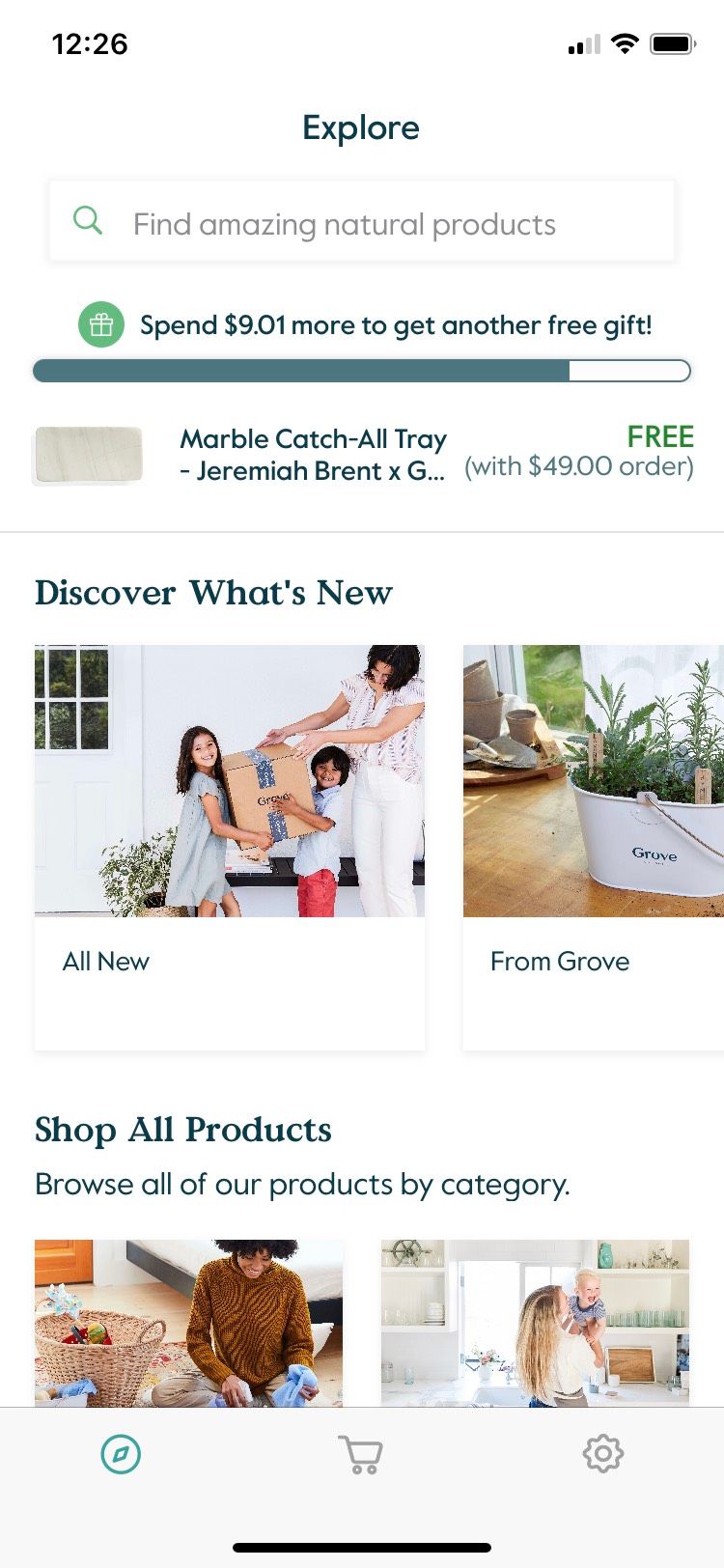This screenshot from a cell phone displays the interface of a shopping app. In the top right-hand corner, icons indicate a full battery, full Wi-Fi connection, and two bars of cellular service. The top left shows the time as 12:26. The page is titled "Explore," and features a search bar with a green magnifying glass icon and the prompt "Find amazing natural products." 

Below the search bar, there is a green circle with a white package icon accompanied by the message, "Spend $9.01 more to get another free gift." A blue progress bar beneath this message is nearly full. Below, an image of a marble catch-all tray is displayed with the caption, "Marble Catch-All Tray by Jeremiah Brent, free with $49 order."

Further down, the section titled "Discover What's New" features two images. On the left, a boy, a girl, and a mother are carrying a package together, labeled "All New." On the right, an image showcases indoor houseplants in a stylish white bucket with the note "From Grove."

At the bottom, the section "Shop All Products" invites users to "Browse all of our products by category." This is accompanied by two images: one on the left shows a woman cleaning something on the floor, and on the right, another woman holds up a baby in a kitchen setting.